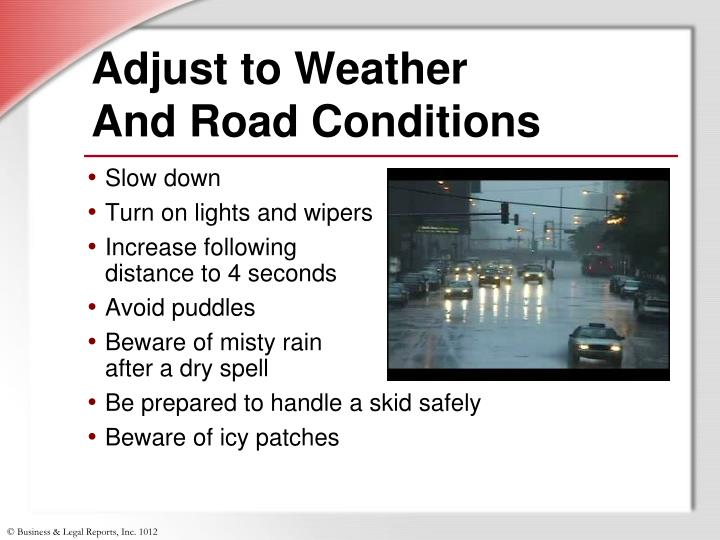This detailed PowerPoint slide is designed to instruct viewers on how to safely adjust to various weather and road conditions. It features a sleek, modern white background framed with a gray border that fades into white at the lower left corner. Dominating the top left corner is a red triangular decoration that adds a pop of color. The title, "Adjust to Weather and Road Conditions," is prominently displayed in bold black text at the top of the slide.

Under the title, a red horizontal separator sets apart seven key safety tips, each identified by a red bullet point and black text. The tips are: slow down, turn on lights and wipers, increase following distance to four seconds, avoid puddles, beware of misty rain after a dry spell, be prepared to handle a skid safely, and beware of icy patches.

To the right of these bullet points, the slide includes a photograph depicting an urban street scene on what appears to be a rainy day. Cars with their headlights on are driving towards the viewer, framed by traffic lights and dimly lit buildings that hint at an early evening or morning setting. The overall ambiance underscores the practical advice provided.

In the bottom left corner of the slide, a small copyright notice reads, "Copyright Business and Legal Reports, Inc. 2012," grounding the image in its authoritative source.